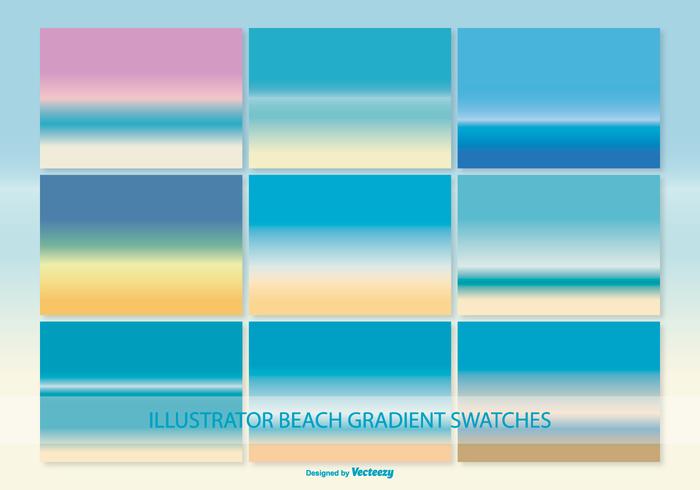This digital image, in landscape orientation, features a grid of nine color illustrations, each representing different beach gradient swatches. Organized in three rows and three columns, each swatch vividly depicts a scene transitioning from shoreline to sky. For instance, in the top left, there is a blend of pink sky, aqua water, and white sand, while the neighboring swatch to the right showcases an aqua sky, light aqua water, and cream-colored sand. The top right swatch illustrates a clear blue sky, white horizon, and dark blue foreground. Each illustration seamlessly captures the essence of a beach scene, with colors ranging from light blue, white, and pink evoking sunrises and sunsets, to gradients of brown and green reflecting sandy shores meeting the sea. 

The image's background is divided into a blue top portion and a white bottom portion, harmonizing with the beach themes portrayed. At the very bottom of the image, there is a transparent horizontal strip overlay with the text "Illustrator Beach Gradient Swatches," and directly below that, in blue text, it reads "Designed by Vecteezy." The swatches, set against this soothing background, capture the tranquil beauty of coastal landscapes through their vivid, gradient color schemes.